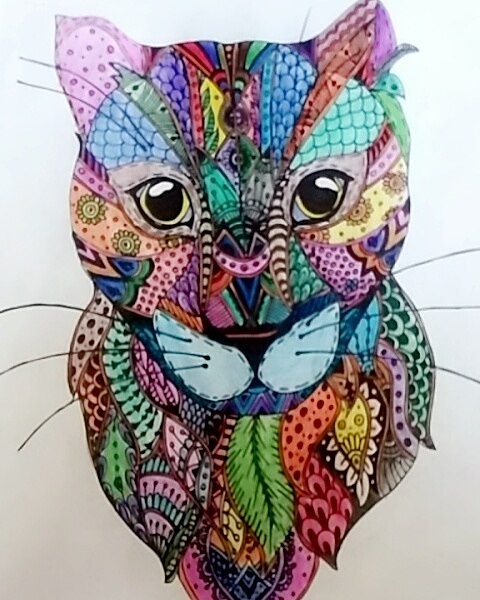This vibrant cat looks more like a decorative artwork due to its myriad of colors. At its center, it features small, wing-shaped circles in blue, with black whiskers extending from this area. Additional black whiskers are found just above its eyebrows. The eyes are solid black, contributing to its striking appearance. The cat’s pattern is richly detailed with floral and nature-inspired elements, featuring bright hues such as green, orange, and red. Its design incorporates sections that resemble butterfly wings in pastel pink and turquoise. Additionally, it has green and yellow patterns adorning its body. The ears are uniquely colored, with one ear in pink and the other in a blend of darker orange and purple. Overall, this cat is a radiant display of mostly bright and lively colors, creating a fun and whimsical appearance.